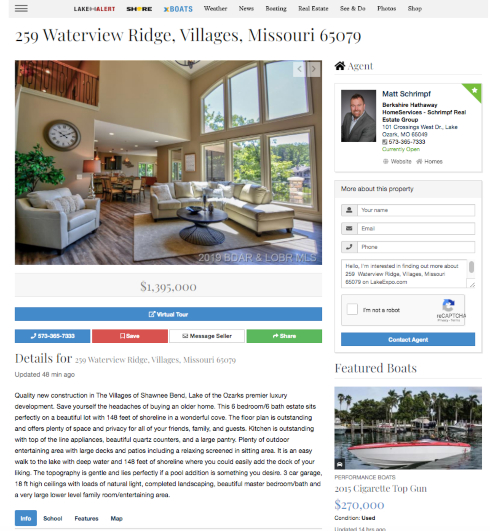The webpage appears to be a detailed real estate listing for a luxurious property located at 259 Waterview Ridge, Villages, Missouri 079. The site features a header titled "Lake H Alert Shore Boats" and offers various navigation options such as Weather, News, Boating, Real Estate, See and Do, Photos, and Shop.

The listing showcases an image from the interior of a grand house described as new quality construction within the prestigious Village of Shawnee Bend, Lake of the Ozarks. Listed at $1,395,000, this estate includes six bedrooms and six bathrooms, set on a beautiful lot with 148 feet of shoreline in a picturesque cove.

The floor plan is lauded for its outstanding design, offering ample space and privacy for friends, family, and guests. The kitchen is highlighted for its top-of-the-line appliances, stunning quartz countertops, and a large pantry. Outdoor entertainment options are abundant with large decks and patios, including a relaxing screened-in sitting area.

The property is described as having easy lake access with deep water suitable for adding a dock, gentle topography ideal for a pool addition, and a three-car garage. Features such as 18-foot high ceilings, loads of natural light, and complete landscaping add to the estate's allure. The luxurious master bedroom, exquisite bathroom, and expansive lower-level family room and entertainment area further emphasize the quality and grandeur of this home.

Additionally, the webpage notes that the realtor representing the property is Matt Shrimp from Berkshire Hathaway HomeServices Shrimp Real Estate Group. Prospective buyers are encouraged to fill out their name, email, and phone number for more information about the property. 

Other sections of the website feature listings for performance boats, such as a 2015 Cigarette Top Gun priced at $270,000, highlighting a range of high-end waterfront lifestyle options available through this real estate platform.